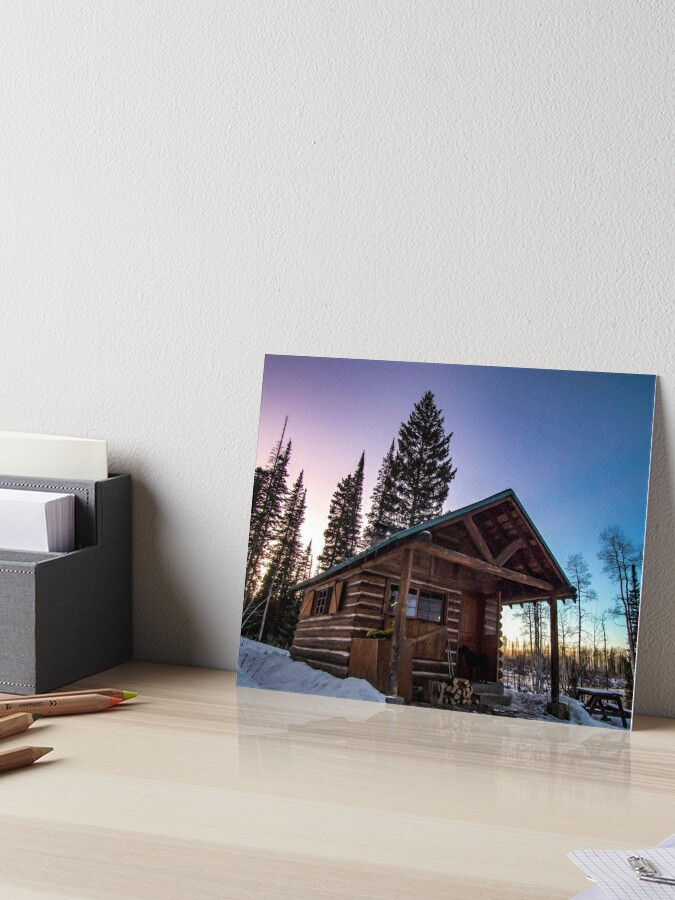The image depicts a minimalist and neatly organized light wood desk positioned against a natural stone-colored wall. At the center of the desk, leaning against the wall, is a high-quality photograph or detailed painting of a log cabin in a snowy, wintry landscape. The cabin appears to be a one-room structure with a tin roof, set amidst towering pine trees under a dreamy sky that transitions from purple to blue, suggesting either a sunrise or early evening light, casting a colorful glow on the scene.

To the left of this striking centerpiece, there is an organizer that holds various papers and cards. On the desk in front of the organizer lay four neatly sharpened, high-quality artist's pencils in colors coral, yellow, gray, and possibly white or blue. Scattered near the pencils are some loose sheets of paper and at the far right corner of the desk, a small collection of paper clips rests on a piece of paper. The overall scene is clean and tidy, resembling a stock photo template meant for showcasing artwork or prints, potentially on a product page.